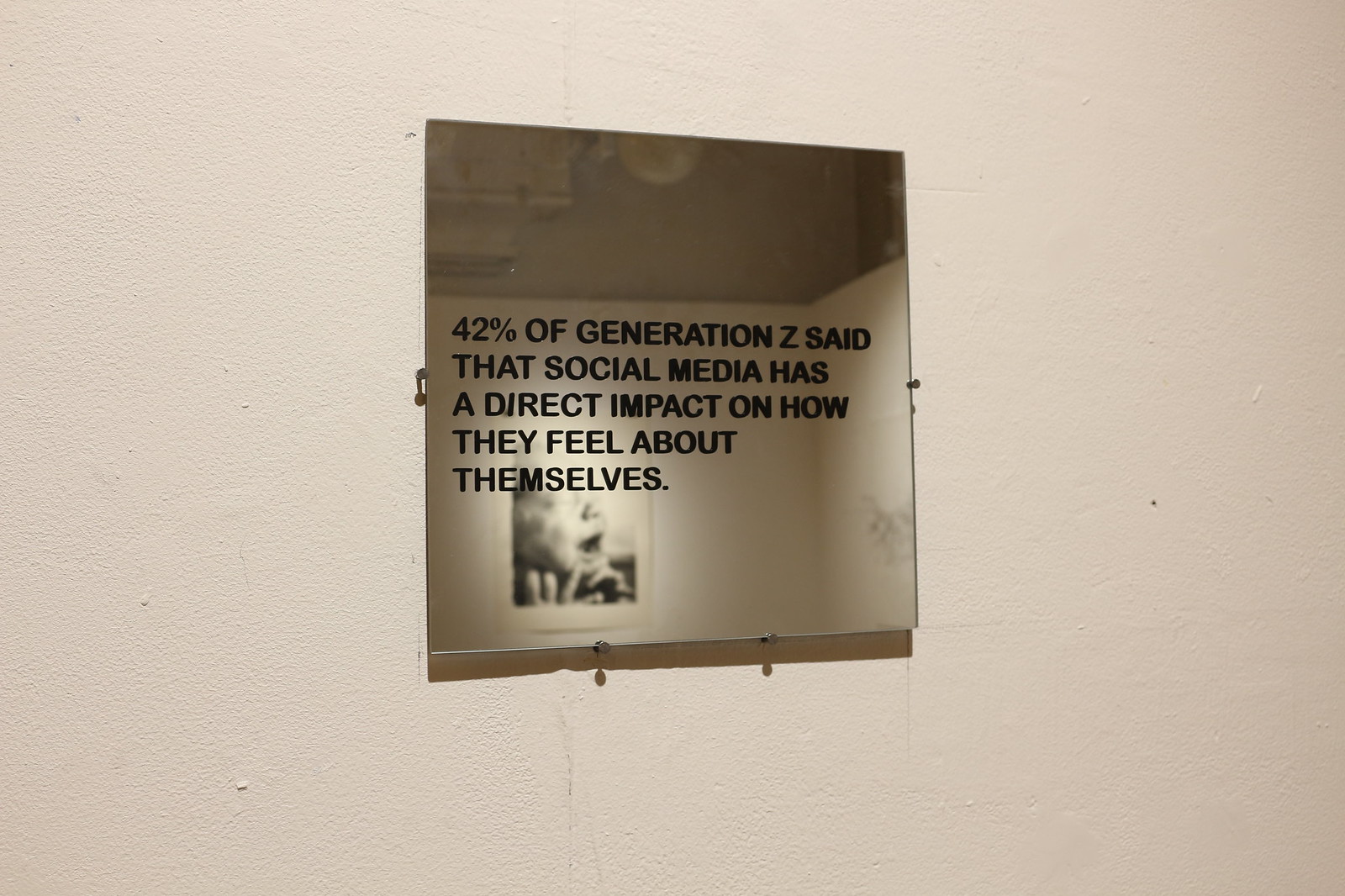This photograph captures an art exhibit in what appears to be an art gallery or museum. Featured prominently is a square mirror mounted on a plain wall, creating a powerful visual and reflective message. The wall is a neutral backdrop, possibly brown or white, adding to the minimalist aesthetic of the display.

Etched onto the mirror is the poignant message: "42% of Generation Z said that social media has a direct impact on how they feel about themselves." This statistic encourages viewers to examine their own reflections and consider the effects of social media on self-perception, effectively turning the observer into a part of the artwork.

In the mirror's reflection, another framed image catches the eye—this time, a photograph of a very young baby with an open mouth and a hand near the face, almost Polaroid-like in its simplicity. Screws securing the mirror and the reflective image of the baby highlight the intentionally sparse and thought-provoking setup. This composition underscores the theme of self-image and the pervasive influence of social media on personal identity, inviting viewers to engage in a moment of introspection.